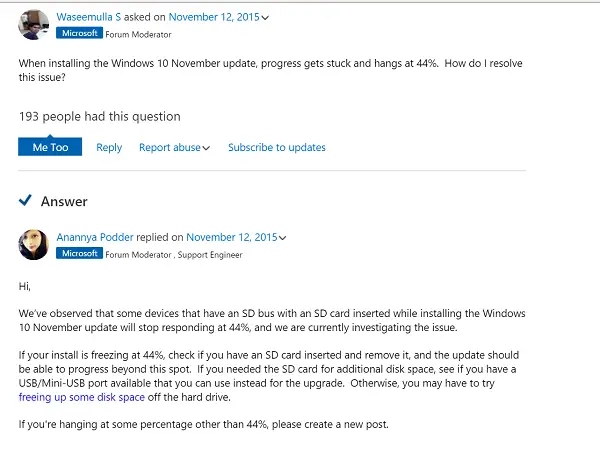In this image, we see a screenshot with a solid white background. The post is by Wasimula S., dated November 12, 2015. The screenshot features a blue button labeled "Microsoft Forum Moderator."

The main content of the post reads as follows: "Here's an image of a young man sitting at a desk. When installing the Windows 10 November update, the progress gets stuck and hangs at 44%. How do I resolve this issue?" This problem is highlighted by the fact that 193 people had the same question.

Below the post, there is a reply from Ananya Potter, a young woman, who is identified as a Microsoft Forum Moderator and Support Engineer. She replied on November 12, 2015, stating: "Hi, we've observed that some devices with an SD bus and an SD card inserted during the installation of the Windows 10 November update will stop responding at 44%. We are currently investigating this issue. If your installation is hanging at a percentage other than 44%, please create a new post."

The detailed descriptions and timestamps provide a clear depiction of the issue at hand and the initial support response from Microsoft.